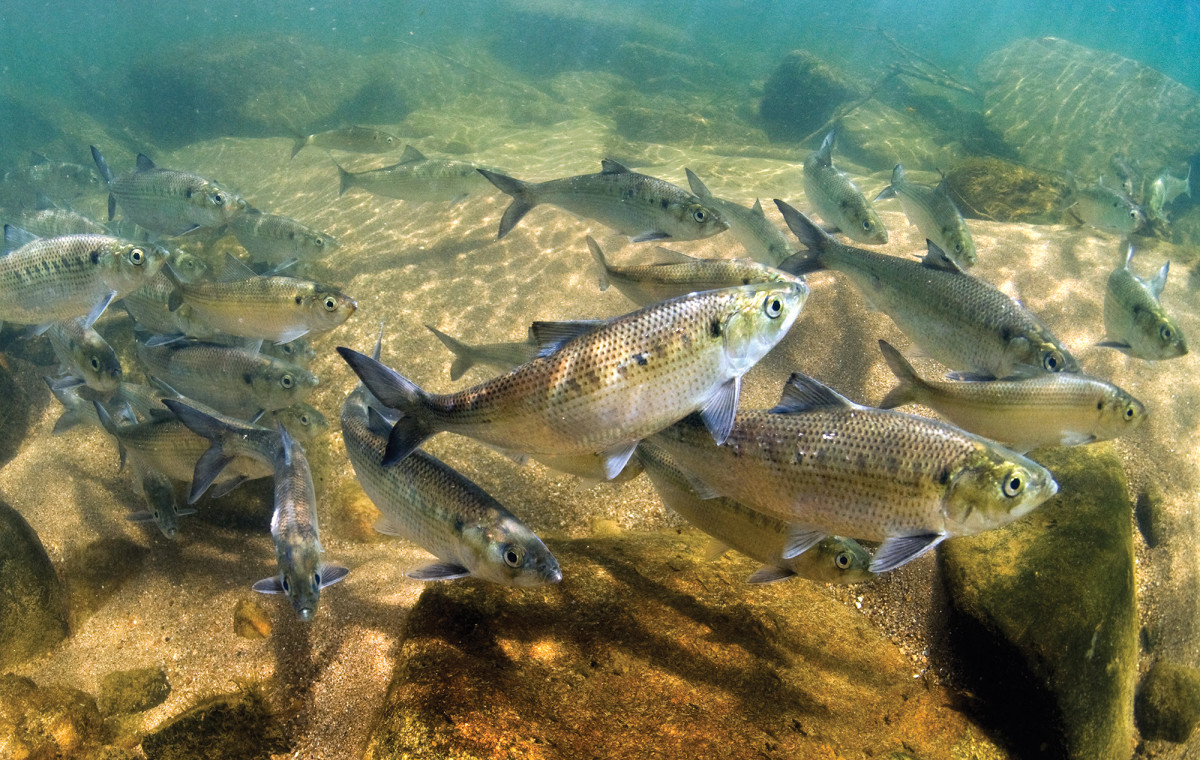The image captures a vibrant underwater scene, possibly viewed through a window of an aquarium or taken with an underwater camera. A school of silver fish, resembling rainbow trout, swims together from the left to the right side of the frame. These fish feature distinct greenish stripes down their backs and faint pink hues, with black spots dotted along their tails and spines. Each fish has one dorsal fin and two ventral fins, and they possess black eyes. The water is a striking greenish-blue, illuminated by sunlight that filters down to a sandy bottom. Scattered rocks of various shapes and sizes provide hiding spots for the fish, and some debris is visible in the background. The bottom left corner shows a concentration of fish, highlighting their uniform appearance despite slight variations in size. The scene is vibrant, showing a harmonious underwater ecosystem.